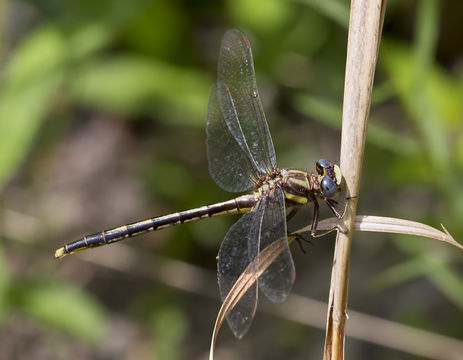The image captures a detailed, close-up shot of a dragonfly perched on a vertical, tan-colored stem amidst an outdoor setting with a blurry green foliage background. The dragonfly is the central focus of the photograph, its head positioned to the right and its long, slender body extending to the left. The body of the dragonfly features a striking pattern of black and yellow markings, culminating in a yellow-tipped tail. Its wings, which are translucent with faint hints of blue, are clearly visible, with two positioned above and two below the insect's body. The dragonfly's prominent black eyes and several legs gripping the stem add to the intricate detail of the image. The background hints at additional branches and leaves, reinforcing the natural environment surrounding this captivating insect.